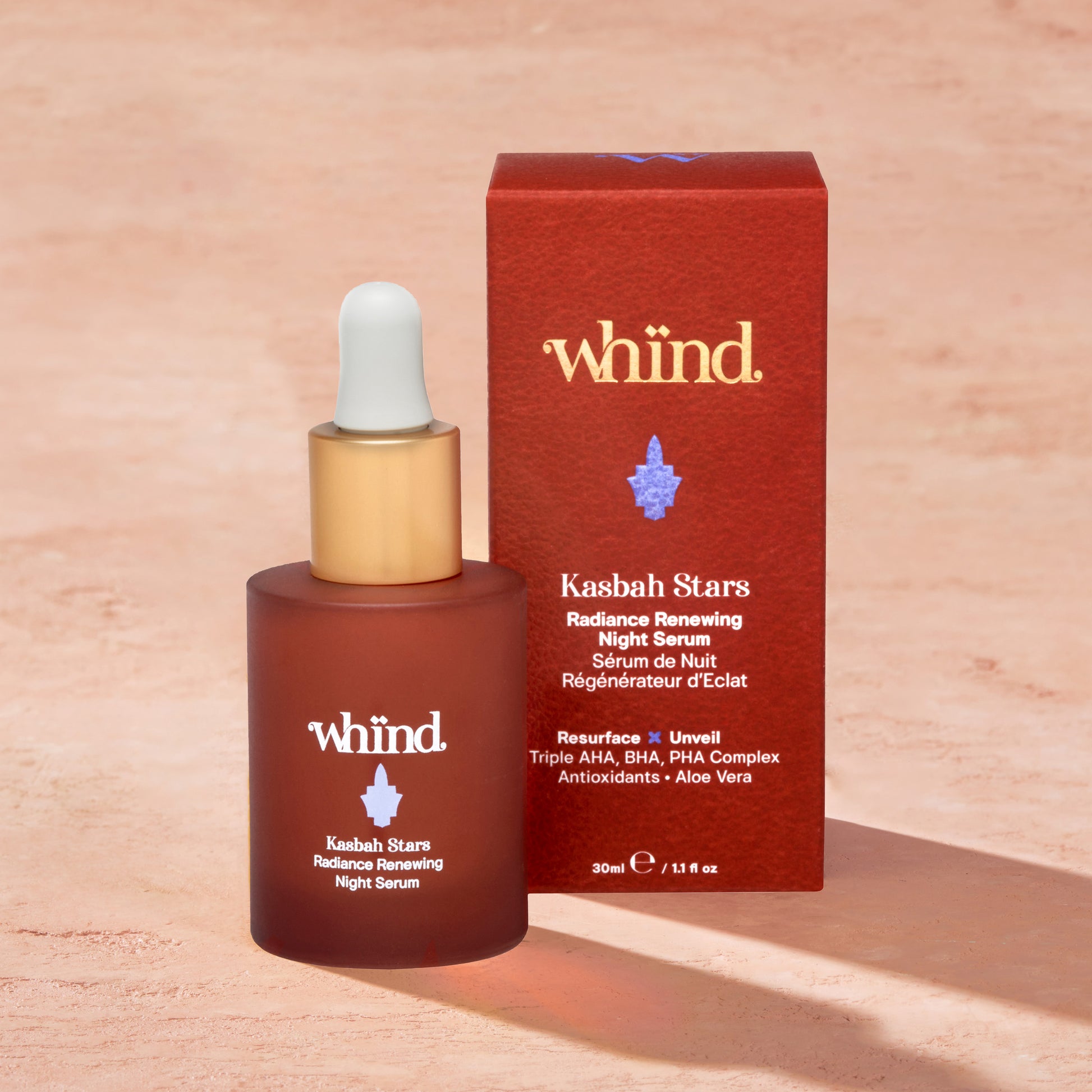The image features a product and its packaging prominently displayed against a peach-colored background. The product includes a burnt orange, dark red bottle with a twistable golden lid. The bottle is labeled with "WIND" (W-H-I-N-D) and a blue emblem resembling a flower underneath it. The text on the bottle reads: "Cosbah Stars Radiance Renewing Night Serum."

Next to the bottle, there is a box, also primarily red, detailed with gold lettering at the top that matches the text on the bottle, "WIND" (W-H-I-N-D), and the same blue flower emblem. The full text on the box includes "Cosbah Stars Radiance Renewing Night Serum," followed by French text: "Serum de Nuit, Regenerator d'Eclat." Below this, the box further details the product's features: "Resurface, Unveil, Triple AHA, BHA, PHA Complex, Antioxidants, Aloe Vera." At the very bottom, the box denotes the product's size: "30 mL / 1.1 fl oz."